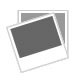The image showcases a modern professional photograph of a detailed maritime navigational sextant made of shiny, intricate brass. It features a semicircular scale with an arm that swings to measure angles, as well as several mirrors or filters that can be adjusted depending on lighting conditions and a telescope for observing celestial bodies. The sextant is perched atop its storage box, crafted from dark and light grained wood with brass fittings and black hardware, including clasps and a handle. The box also bears the logo 'Varth, V-A-R-T-H' on a tan background. The setting is against a light blue striped, ribbed surface that resembles waves of sand, adding to the image's intricate and ornate aesthetic.